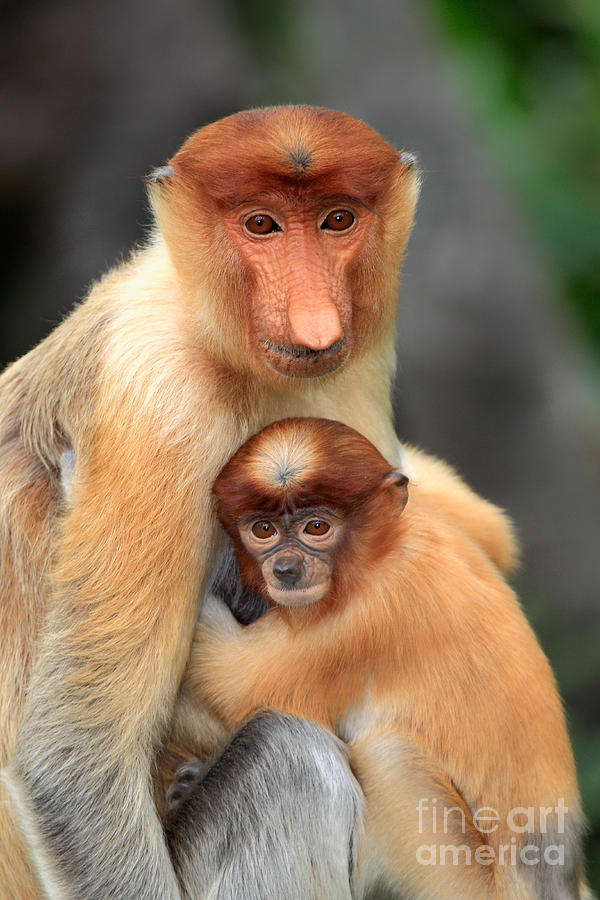The outdoor color photograph is a striking close-up of two red-faced monkeys, likely a mother and her baby. The frame is completely filled with these creatures, emphasizing their intricate details and fostered connection. The monkeys are primarily light yellowish-tan with reddish-brown heads and distinct dark brown eyes. The mother's face is prominently pinkish, free of fur, with a characteristic long, light pink nose that distinguishes her as a proboscis monkey. In contrast, the baby's stubby, darker nose signals youth. Both display a burnt orange hue on top of their heads, transitioning to a brighter orange on the sides. The background is softly blurred into shades of gray, ensuring the focus remains on the monkeys' expressive faces. They sit hunched, the baby in the foreground gripping the mother's chest and both gazing directly at the camera. The lower right corner features the white text "Fine Art America," hinting at the image's commercial availability as a fine art print or poster.